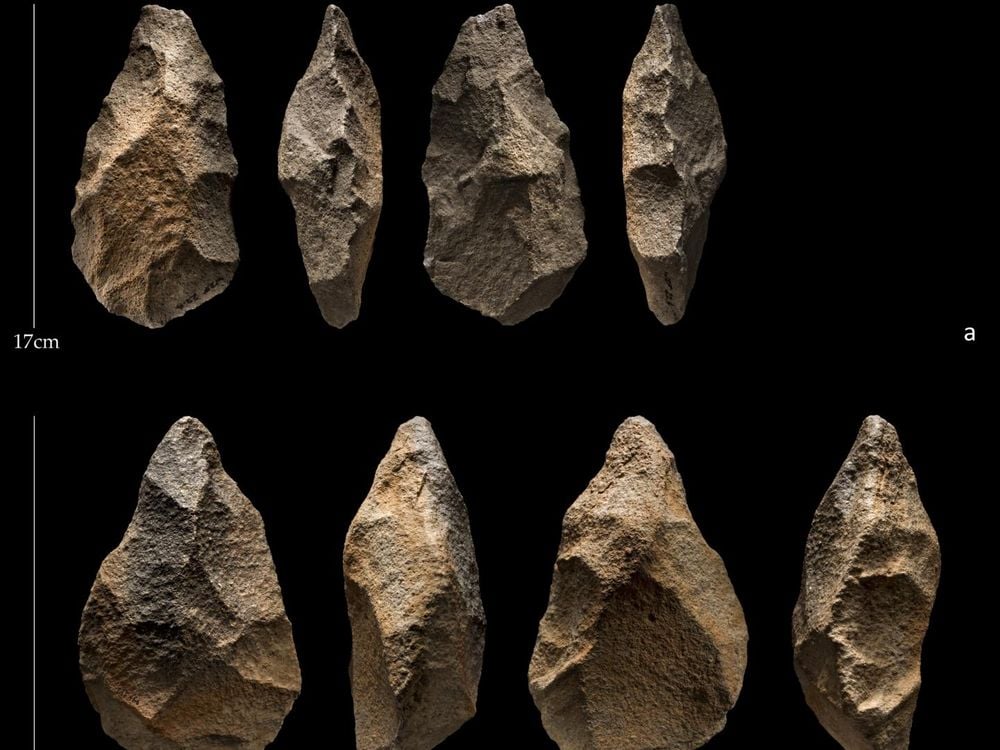This photograph showcases eight ancient stone artifacts, likely used as tools or weapons such as spearheads or arrowheads, meticulously napped to form sharp edges. The artifacts, with a rough stone texture, display a series of small indentations along their edges, indicative of an intentional chipping technique. They are arranged in two neat rows against a black background—four spearheads at the top and four slightly larger ones at the bottom. The stones vary in shades of gray and brown, each forming a pointed end, with some shaped like triangles and others like diamonds. Shadows cast on either side of the stones highlight their rugged folds and ridges. A measurement indicator on the left denotes "17 centimeters," and a small "A" is visible on the right, providing a clear scale for the size of these ancient relics.